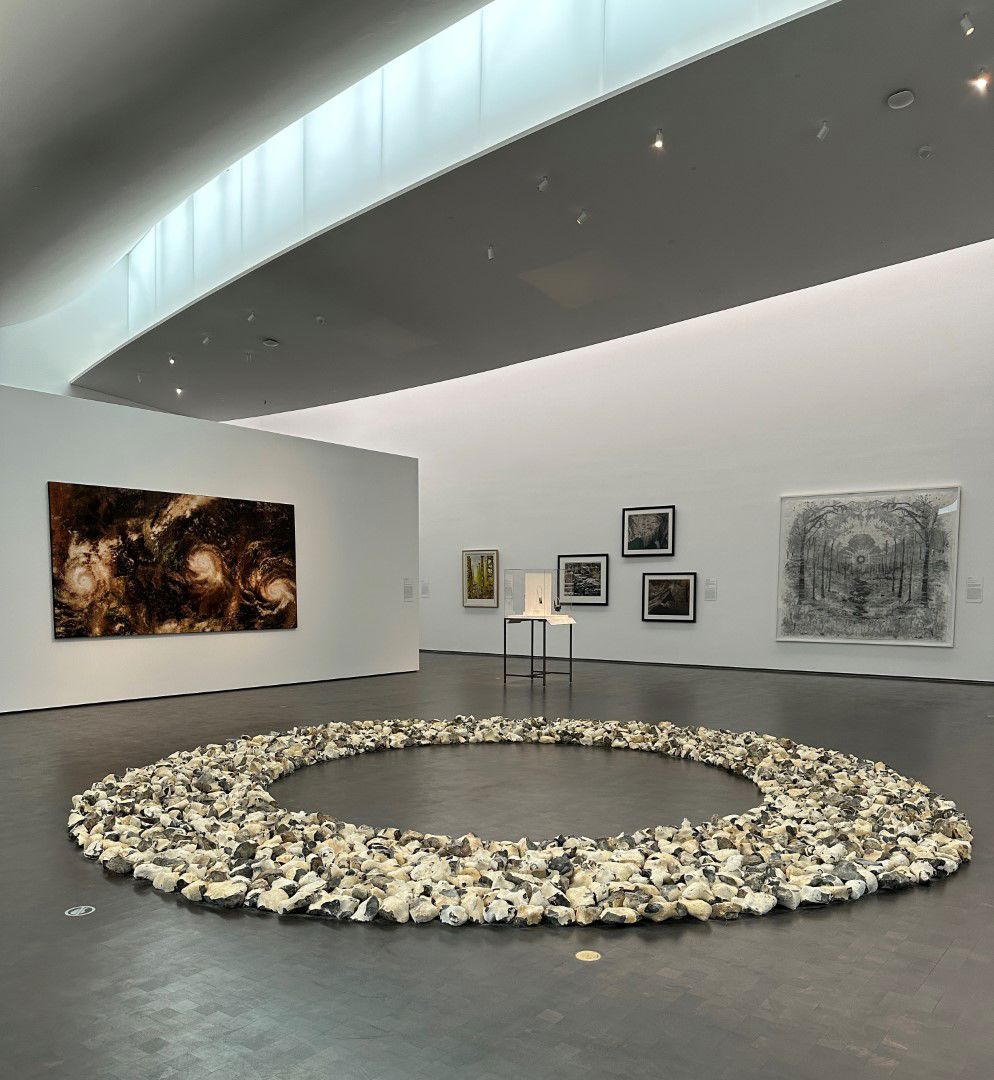The image depicts a striking art installation in a futuristic-looking museum room characterized by its white and grey color scheme. The room has a spacious, minimalist design with white walls and a grey tile floor. Overhead, a skylight or elevated walkway allows light to spill into the space, enhancing the brightness. 

In the center of the room lies the focal point of the installation: a perfectly arranged circle composed of dozens of rocks or ceramic pieces in various shades of grey, white, brown, and tan, resembling a donut with an empty central circle that reveals the grey floor beneath. 

On the walls, several artworks are displayed. To the left of the rock formation, a smaller portrait on a white wall appears to be a cosmic event or hurricane tracker. Adjacent to this, five other photos adorn the wall, including illustrations that resemble a galaxy, trees, and possibly scenes involving cars and lampposts. In the middle of the room, an apparatus on a desk further accentuates the sophisticated, gallery-like atmosphere.